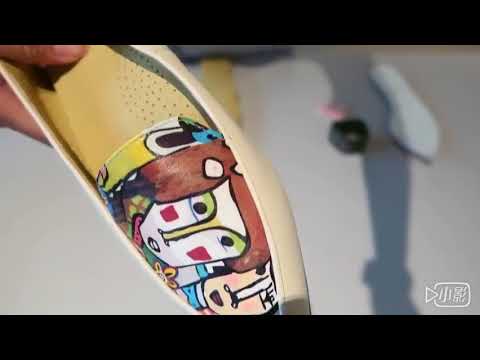The image depicts a scene where a person's brown thumb and forefinger are gripping a small, decorative shoe, prominently centered. The shoe itself is light yellow, possibly a Moccasin type, featuring a colorful, intricate illustration on its top. This illustration portrays two vivid, cartoonish faces: one face has red hair, a long nose, a white complexion, green eye shadow, and red squares on its cheeks; the other face displays dark black eyes, a long white nose, and brownish lips. The colors surrounding the faces include a vibrant palette of blue, yellow, green, orange, brown, pink, and white. The shoe's insole is yellow with ventilation dots. 

The background of the image is primarily white, with black strips bordering the top and bottom. In the backdrop, additional objects can be discerned, possibly another shoe, and there is a faint shadow whose origins are unclear. A logo is located in the bottom right corner, while other ground objects contribute to the setting, which appears to be outdoors in broad daylight, lending an artistic vibe to the scene.